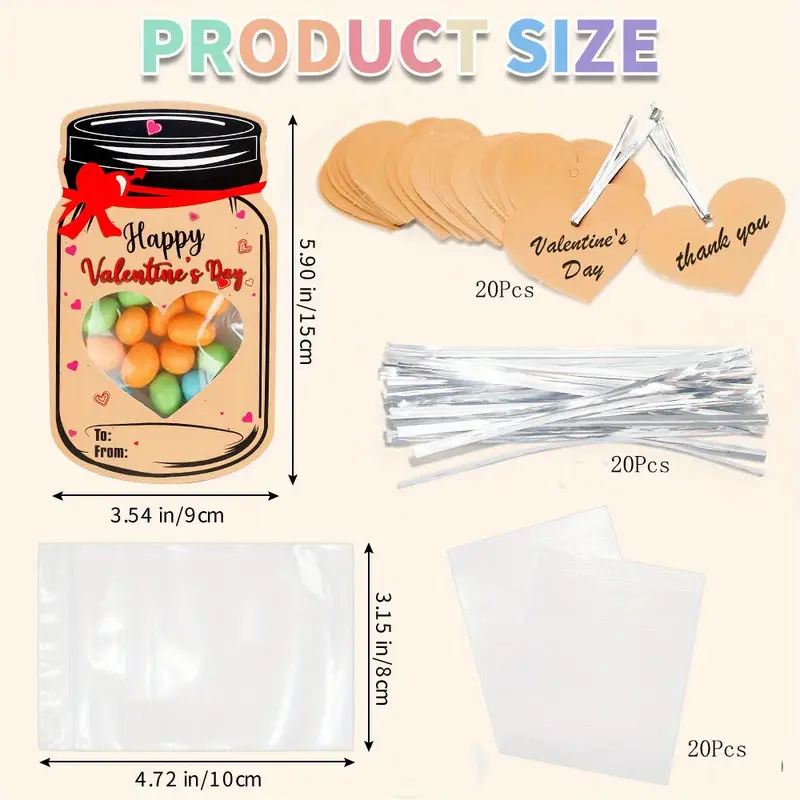The image is a detailed product description poster for Valentine's Day themed gift baggies. At the top, the title "PRODUCT SIZE" is displayed in all capital letters, each character a different color: green, tan, mauve, blue, and purple. On the left side of the poster is an illustration of an orange mason jar with a black top and a red ribbon, labeled "Happy Valentine's Day" with "happy" in black and "Valentine's Day" in red. The jar features a heart-shaped cutout with clear cellophane, revealing candies or jelly beans inside.

To the right, the poster details the dimensions of the baggies: 5.9 inches (15 cm) in height and 3.5 inches (9 cm) in width. Additionally, it includes a diagram with arrows indicating these measurements. On the top right corner, there are heart-shaped tags in a beige-brown color. Some hearts are labeled "Valentine's Day" in black cursive writing, while others say "Thank You." The poster specifies that the package includes 20 heart-shaped tags, 20 silver twist ties, and 20 clear plastic baggies. The poster’s background is a cream color, giving it a simple yet elegant appearance, ideal for highlighting the detailed, colorful product information.